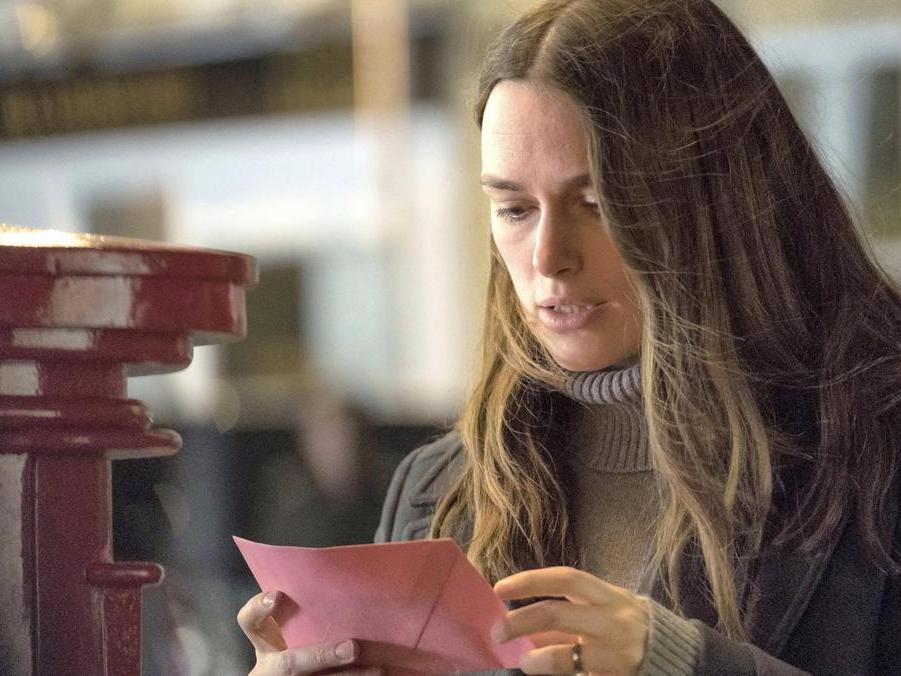This photograph, set in a rectangular frame with the shorter sides on the left and right, captures a Caucasian woman who appears to be around 30 years old. The composition of the image focuses on her from mid-chest up to just below the top of her head, occupying about one-third of the frame. She has light brown, slightly wavy hair that falls just past her shoulders, styled with a mix of side and center parting. 

The woman stands in the foreground, her torso mostly facing the camera with a subtle angle to the right shoulder, creating a dynamic posture. She gazes intently at a pink envelope held in her hands, her expression serious and reflective, suggesting the envelope's contents might be significant or consequential. Her bottom front teeth are visible as she concentrates on the envelope.

Her attire includes a high-necked, light gray turtleneck sweater with vertical ribbing, complemented by a dark gray or gray-brown jacket featuring notched lapels. On her left hand, she wears a gold ring, with both hands engaged with the envelope; the left hand appears to graze its edge.

The background, slightly blurred, hints at an indoor setting, possibly a library, with various indistinct shapes and shelves adding depth to the scene. Prominently on the left side, a series of shiny red metal discs on a post suggest a sculptural element. A secondary smaller post with a cylinder appears beneath it. Additionally, a white, blurry line and shape with sharp angles are visible near the top left, contributing to the cubist-like blur in the background, which includes gray and black tones.

Overall, the photograph portrays a poignant moment of anticipation and reflection for the young woman, all against a backdrop that offers texture without distraction.